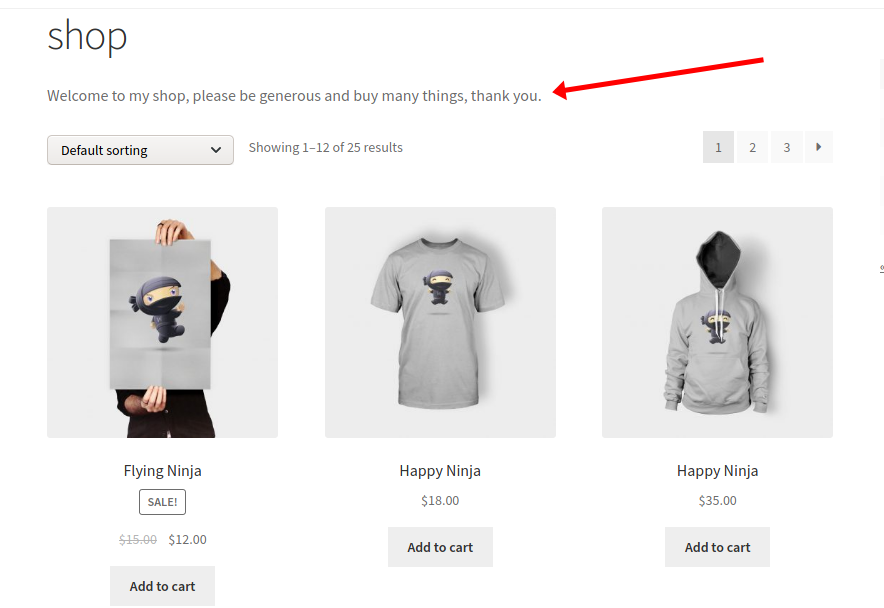The screenshot displays an online shop interface. On the far left, 'Shop' is written in bold black letters. Immediately below, there's a welcoming message that reads, "Welcome to my shop. Please be generous and buy many things," accompanied by a large red arrow pointing to the end of the sentence. Beneath the welcome message is a rectangular gray box with a down arrow indicating a dropdown menu labeled "Default sorting." Alongside this, there is a note stating, "Showing 12 of 25 results."

To the far right are navigational controls for the shop. A series of small gray boxes numbered one through three, along with a forward arrow, signify the current page as the first page of results.

The product listings feature various t-shirts, including one called "Flying Ninja." This character is depicted in all black with only its eyes visible and a small propeller attached to its back, suggesting it is flying. The Flying Ninja t-shirts are on sale. Another product, the "Happy Ninja" hoodie, also shows only the eyes of the ninja and is dressed in all black. The Happy Ninja t-shirt is priced at $18, while the hoodie costs $35. Each product listing includes an 'Add to Cart' button below the price.